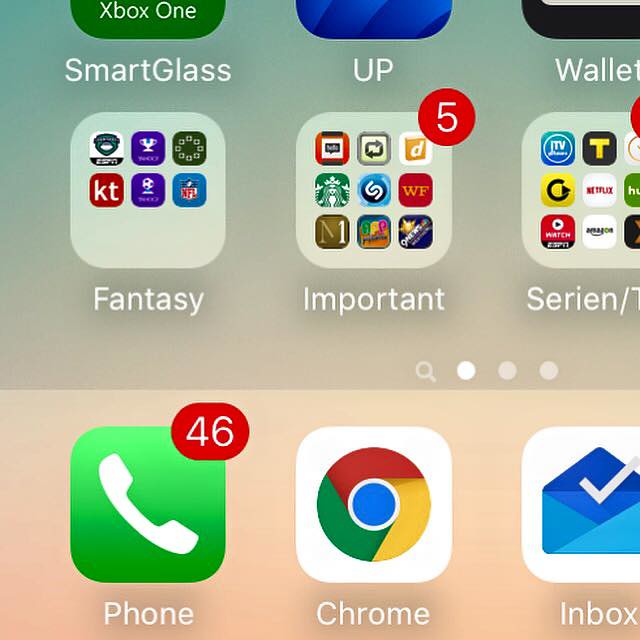A detailed descriptive caption for the image could be:

"This screenshot features a mobile phone home screen in a three-by-three grid layout, with nine visible apps. The top row includes 'Xbox One SmartGlass' with its distinguishable green and white logo, an app with a blue logo titled 'Up', and another app with a black icon labeled 'Wallet'. The second row hosts a folder named 'Fantasy' containing six app logos for services such as Yahoo Fantasy and NFL. Adjacent to it is a folder named 'Important', holding nine icons including banking apps like Wells Fargo. To the right of 'Important' is a folder labeled 'Syrian/TV' housing streaming apps like Netflix, Hulu, and ESPN Watch. There are ellipsis (three dots) indicating more apps can be accessed by scrolling. At the bottom of the screen, three permanently fixed apps reside: 'Phone', 'Chrome', and 'Inbox'."